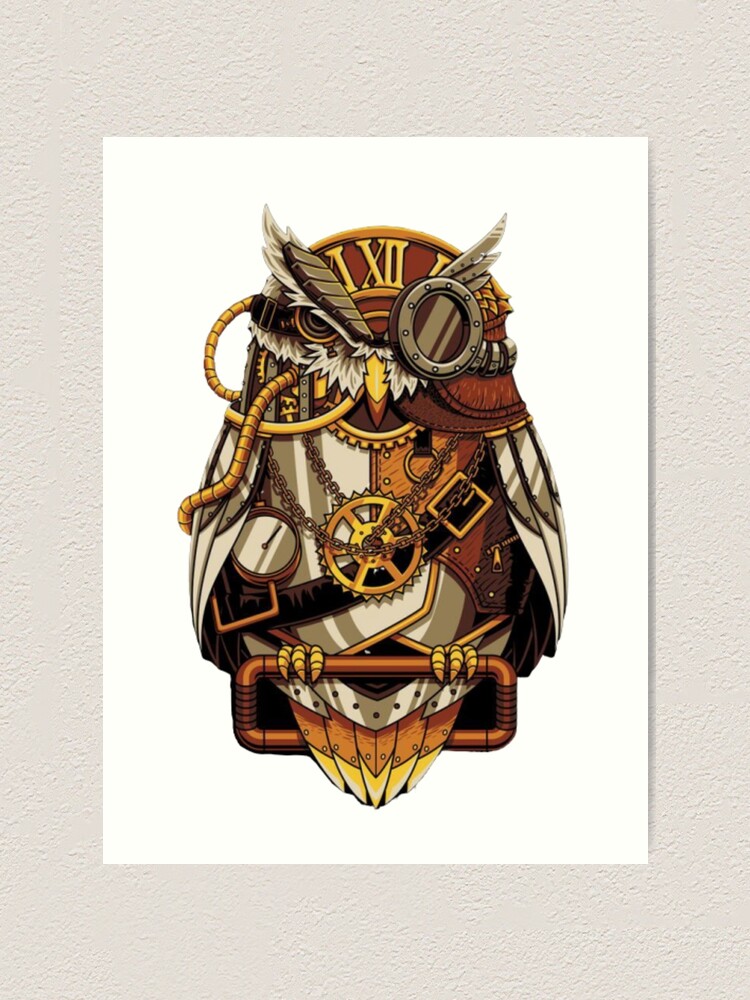The image depicts a meticulously detailed steampunk owl illustration, captured in a drawing or painting style. The owl features a prominent yellow eye and a monocle resembling a ship's porthole over its other eye. The eyebrows are fluffy gray and brown feathers, accented by Roman numerals I, X, and XI above its head. Encompassing its head and body are various steampunk elements, including ropes, cords, and golden tubes that protrude from the head and exit towards the back. A complex array of gears with chains wrap around the owl, adding to its mechanical aesthetic. The owl dons a leather vest with gold buckles and chrome attachments, while its small talons rest on a bronze pipe base. The feathers around its neck and body exhibit a fusion of colors, transitioning from white metal to orange and yellow shades. The tail feathers appear jointed and riveted, reflecting a mix of chrome and golden hues. Around its neck, there is a chain holding up a gold cogwheel like a necklace, enhancing its grandiose steampunk appearance. All these intricate details are set against a white background, taped to a white stucco-like wall.